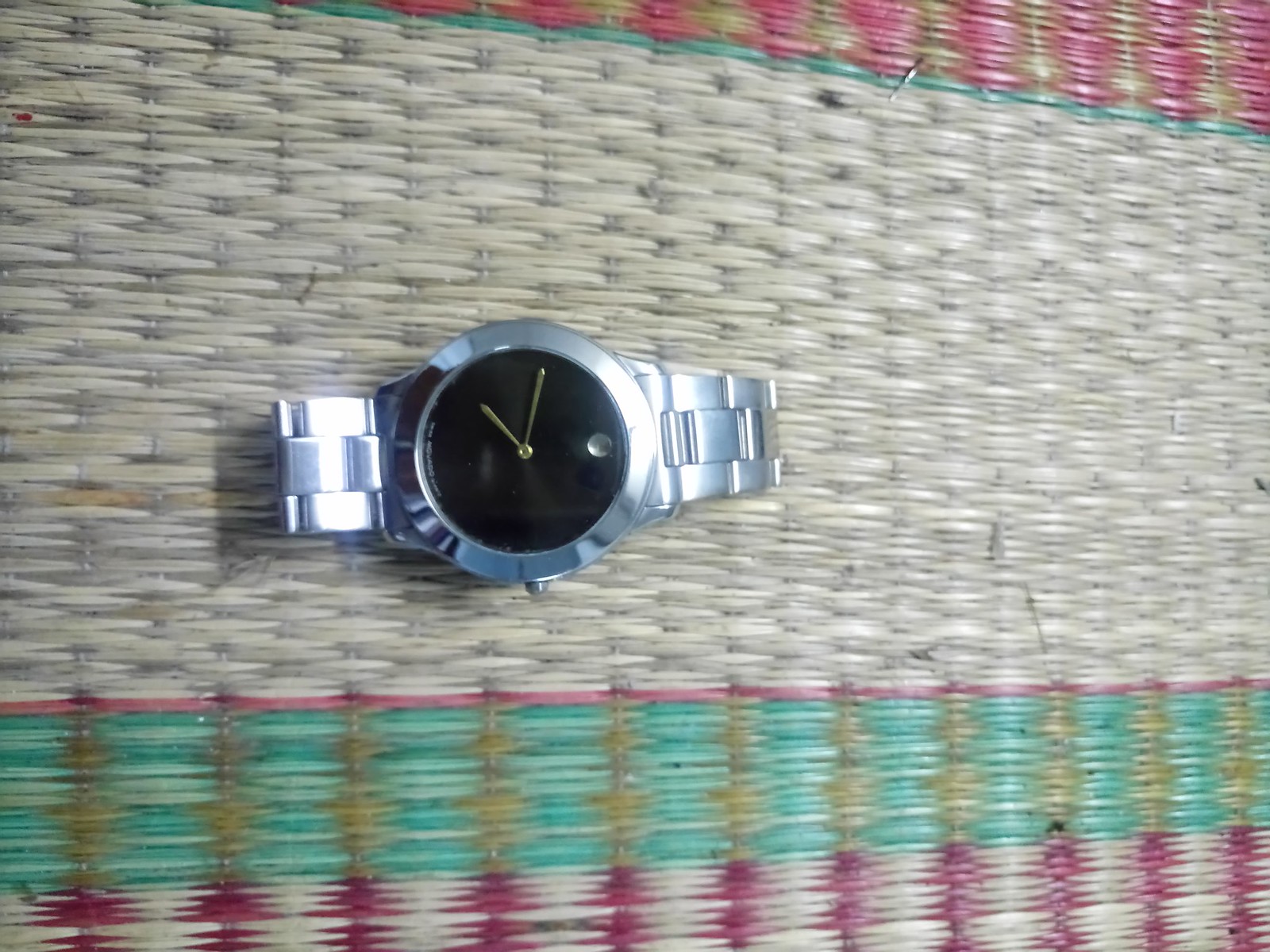This color photograph captures a sophisticated analog wristwatch placed atop a beautifully woven fabric surface. The fabric exhibits a rich tapestry of colors and textures, featuring a central silver-gray band that exudes elegance. At the top of the fabric, a striking stripe combines gold with a subtle rose-pink hue, creating a gentle contrast. Below this, a captivating turquoise blue and gold stripe adds a pop of color, followed by a delicate lavender and white stripe further down.

The wristwatch itself is a masterpiece of silver-toned metal craftsmanship. Its round frame and matching watchband showcase an understated yet refined aesthetic. The stark black face of the watch is minimalist, eschewing numbers for simplistic elegance, and is complemented by sleek gold minute and hour hands. The time displayed on this classic timepiece is precisely five minutes past eleven.